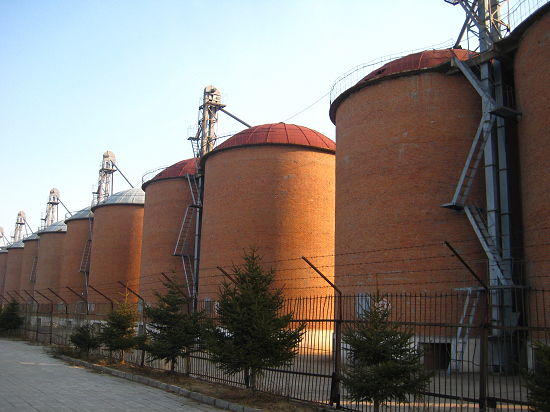This image features an outdoor scene showcasing approximately eight or nine silo-like structures made from terracotta-colored stone, giving them a reddish-brown hue. These large, rounded buildings are arranged in pairs and are topped with red curved roofs that resemble an umbrella shape. Each silo has ladder stairs, or a stairway, extending up to the top and connecting to a sloping mechanism for loading into the storage unit. 

The entire row of silos is situated behind a black wrought iron fence adorned with four layers of barbed wire, clearly designed for security. The fence is flanked by gray pavement along a road. Small green trees are visible at the base of the fence, adding a touch of nature to the industrial setting. The background of the image is a blue sky that transitions from a darker shade on the upper left to lighter hues as it moves toward the center.

Between the silos, gray piping and cranes are noticeable, indicating an area built for functionality. The silo tops toward the back of the image appear to be white, distinguishing them from the red roofs of the ones in the forefront. This detailed scene captures the essence of an industrial storage area with a touch of natural elements and a secure perimeter.